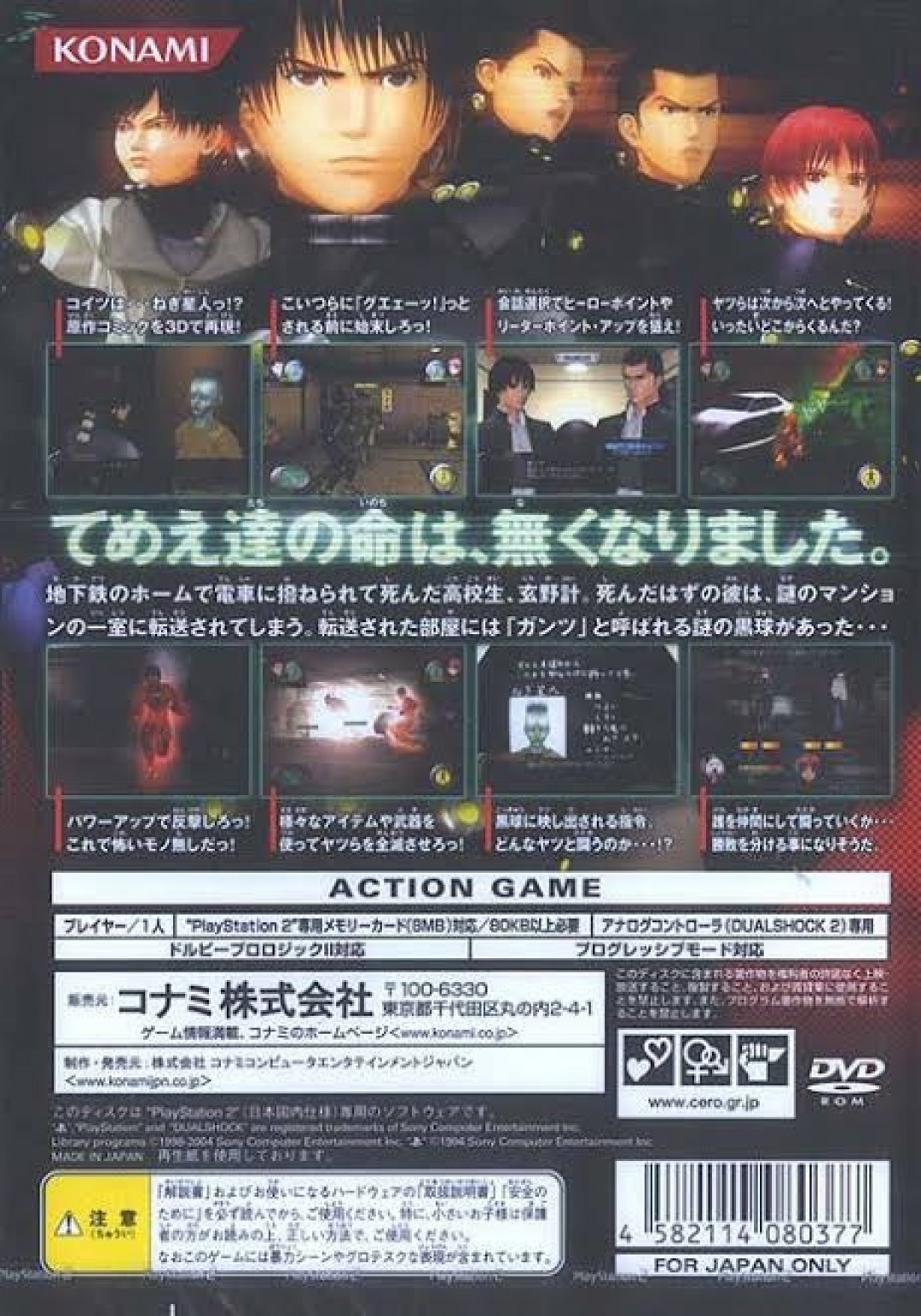This detailed image depicts the back cover of a PlayStation 2 era video game DVD-ROM from Konami, designed for the Japanese market. Dominating the upper section are five animated characters in a stern, scowling disposition. These characters include four males—three with dark hair and one with red hair—and a female with dark hair, all gazing in different directions. The Konami logo is prominently featured in white font on a red ribbon in the top left corner.

Beneath these characters, there are two rows of four rectangular gameplay screenshots, eight in total, depicting various scenes from the game. Most of the cover is cluttered with Japanese text, rendered in a mix of whitish-green and white colors, detailing the game's specifications and features. The only English text visible includes the Konami logo and the words "Action Game." A barcode is located in the lower right corner, accompanied by a "For Japan Only" statement, along with DVD and PlayStation compatibility symbols. The dark-toned background accentuates the vivid design elements, making the package a definitive example of video game box art.